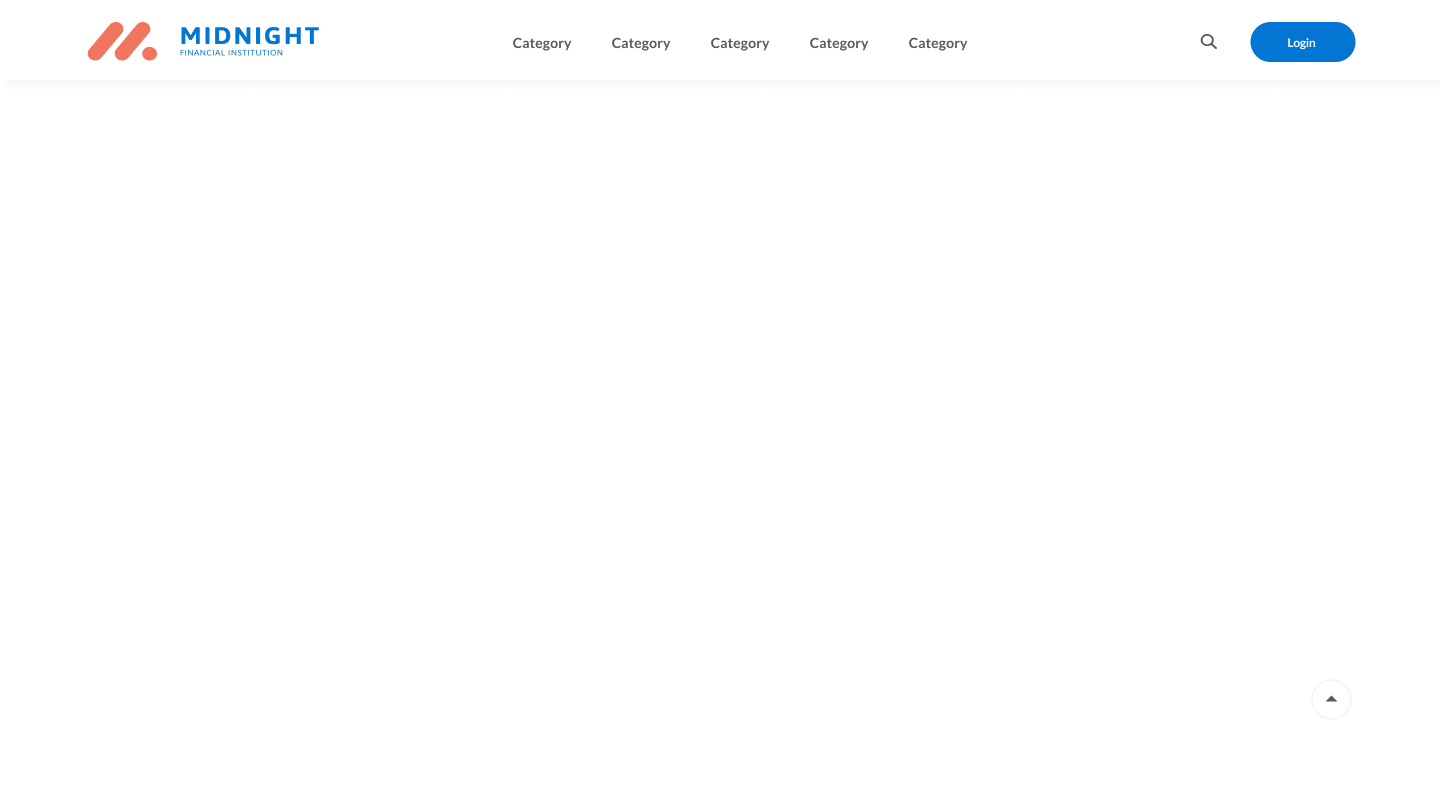The image showcases a partially loaded webpage, appearing mostly empty and slightly zoomed out. Dominating the content is a central logo consisting of two slanted, salmon-colored lines intersected by a red circle. Below this logo is the word "MIDNIGHT" in mid-toned, slightly bright blue, written in all caps.

Underneath the title, there are a couple of smaller blue words, but they are too blurry and the view is too zoomed out to read them clearly. To the right, there is a series of five sub-menu items in gray, each labeled "Category" with a capital "C."

Further to the right, there is a slightly pixelated gray magnifying glass icon, indicating a search function. Next to this is a blue, almost oval-shaped button with white text that reads "Login," with a capital "L." Directly below these elements is a thin gray line that spans the page.

Towards the bottom of the image, there is an isolated white circle containing a small gray upward arrow. Apart from these elements, the page lacks additional images or content, highlighting its unfinished or partially loaded state. The quality of the image is decent, though it would benefit from being more zoomed in to better capture the smaller details.